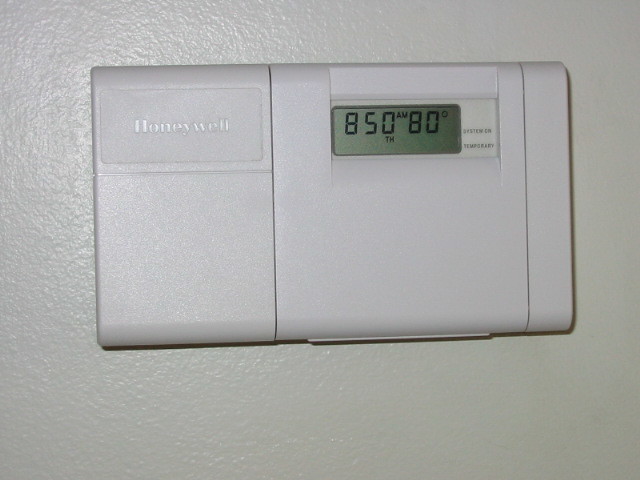In this image, we see a close-up of a Honeywell security system or thermostat mounted on a white wall. The device is a white rectangular unit, divided into three distinct sections. On the top left of the device, the Honeywell logo is prominently displayed. The central section features a small screen displaying "8:50" with "TH" under the zero, suggesting the time, and "80° AM" to the right, indicating the current temperature setting in degrees Fahrenheit. Below the screen, there is a panel that appears to be openable, likely concealing the buttons for adjusting the temperature and other settings. The bottom section is a thin, plain white rectangle that serves to connect the other sections and integrate the device into the wall mount. The pristine white background wall creates a minimalist and clean aesthetic around the device.